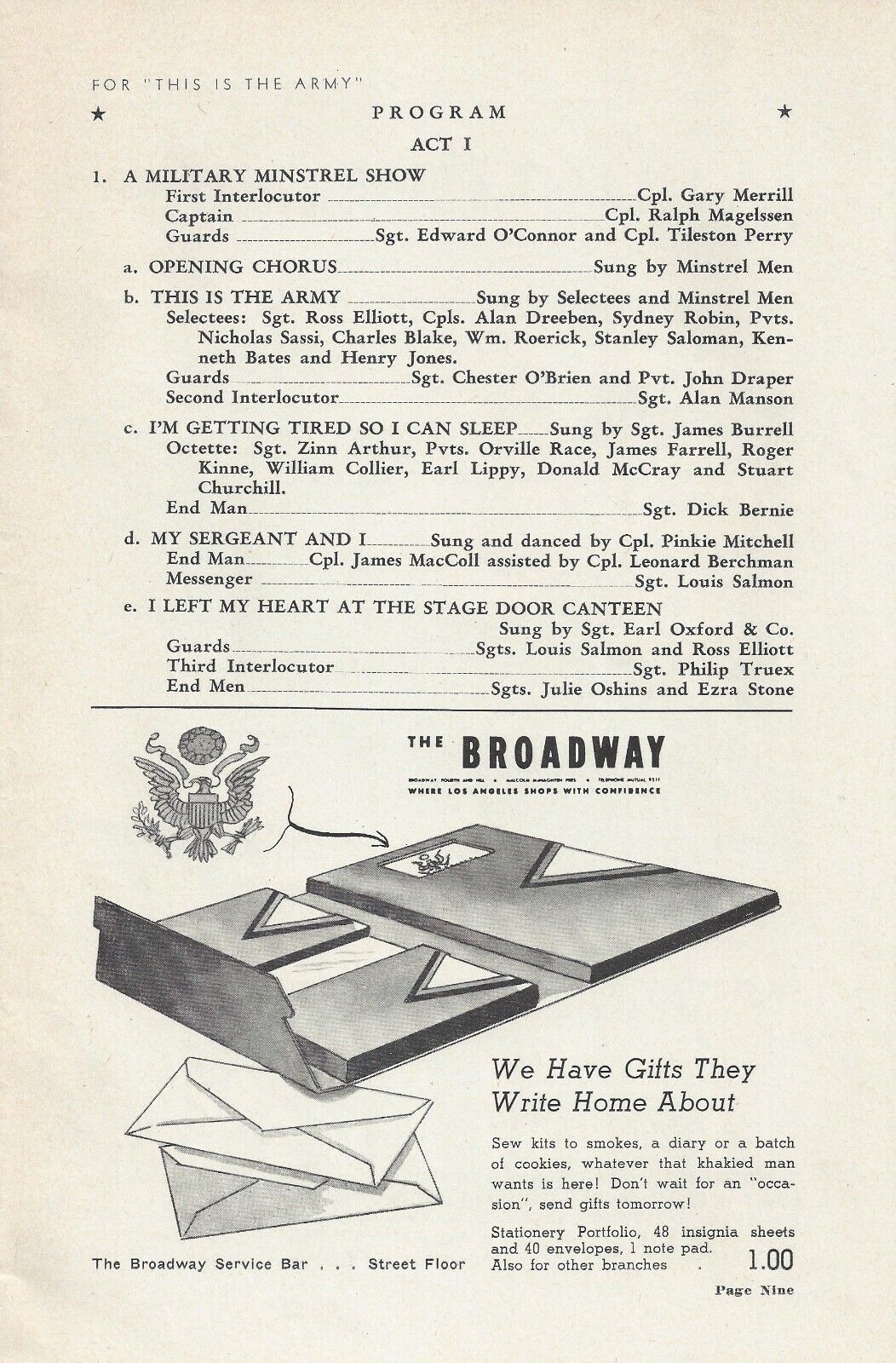The image depicts a vintage program sheet from a Broadway production titled "This is the Army." The program outlines Act One, which is described as a military minstrel show. At the top, the header prominently features the phrase "For 'This is the Army.'" Below that, the program lists various acts and performers, starting with Corporal Gary Merrill as the first interlocutor and Captain Guards, who sings the opening chorus. The detailed cast list includes numerous names and song titles such as "My Sergeant and I" and "I Left My Heart at the Stage Door Canteen." The bottom of the page features an advert with the text "The Broadway, where Los Angeles shops with confidence," and includes the tagline "Gifts They Write Home About." The page also appears to be marked as page 9 of the program, indicating it's part of a larger booklet.